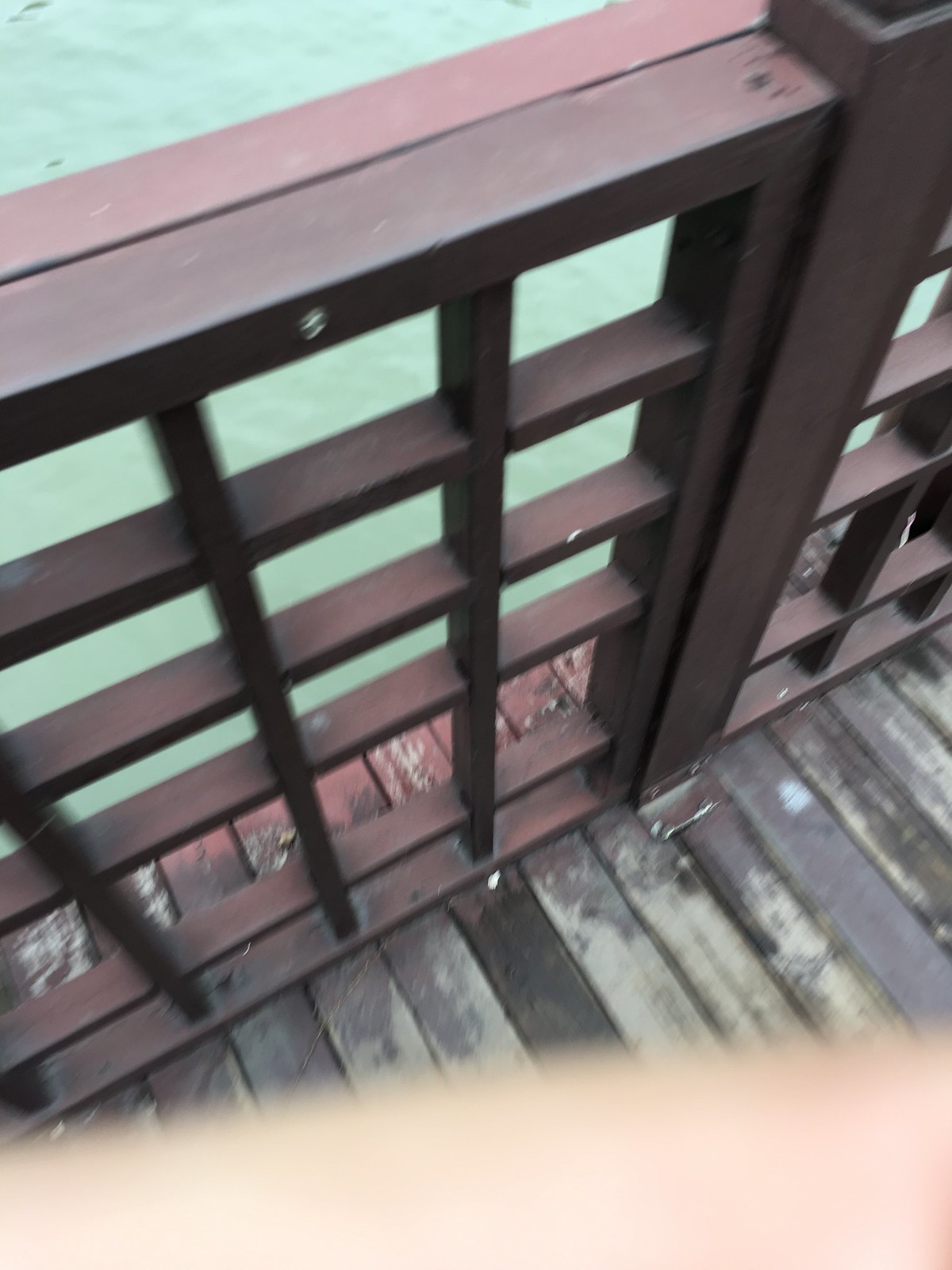The image depicts a wooden dock or boardwalk with a metal fence that has a dull, slightly reddish-brown, grid-like design featuring vertical and horizontal poles. This fence serves as a barrier for safety over the greenish water that occupies the top half of the image. The dock itself consists of wooden planks in varying shades of grey, red, and black, with the lighter wood suggesting well-maintained sections. The sun appears to be shining from the top right, casting a lighter hue on that part of the photo. In the bottom part of the image, there's a blurred section, likely a finger or hand, suggesting someone was taking the picture and inadvertently captured part of their own hand.